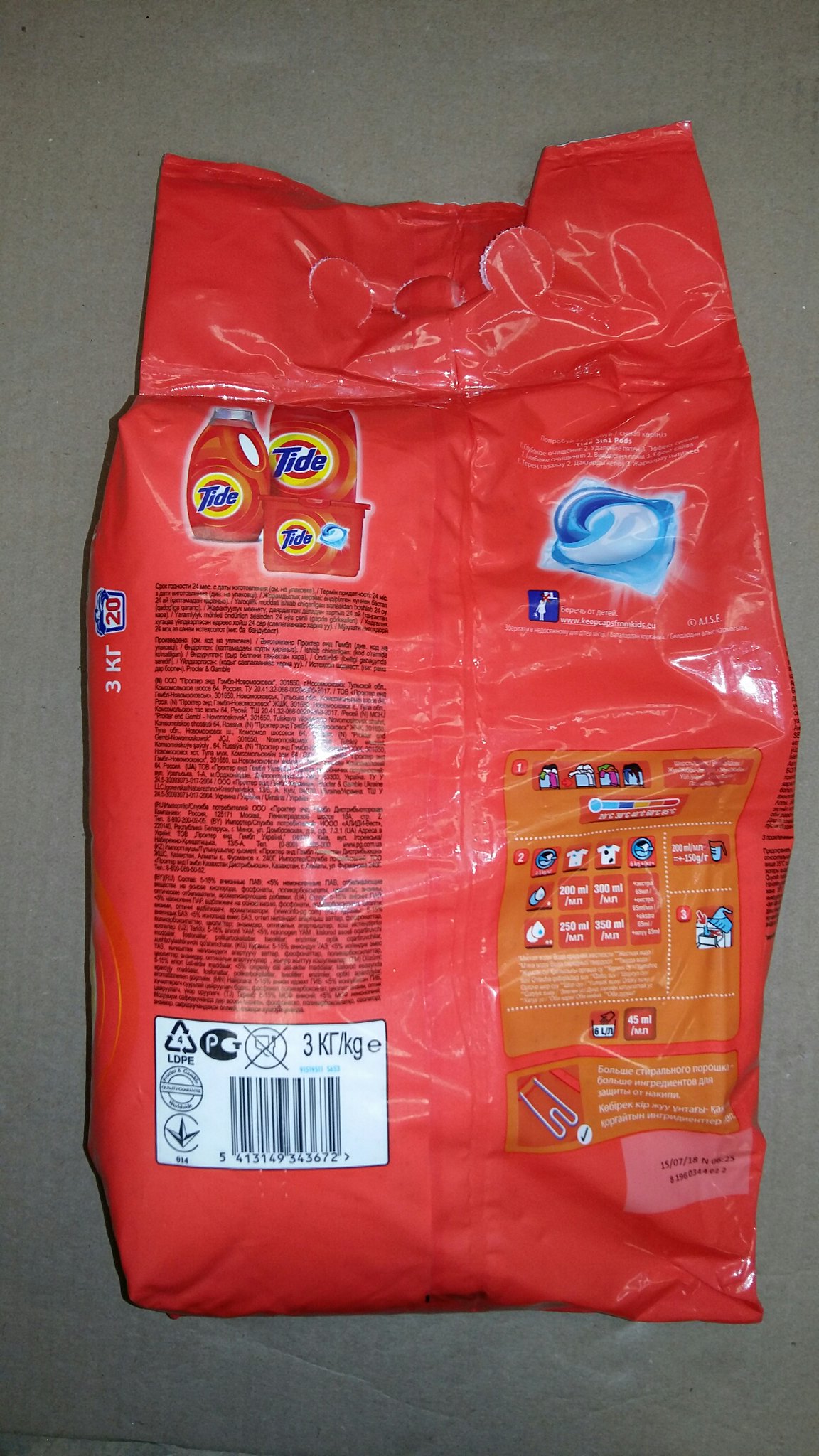This is a color photograph that prominently displays the back of a red bag, likely containing a household product, potentially a laundry detergent refill. In the upper left-hand corner of the bag, there are images of boxes, possibly labeled with "dads" in a very dark blue font, suggesting some association with a brand or specific product line. Adjacent to the boxes, on the right side, there is a blue logo or image resembling a tidal wave, which may indicate the product's association with cleanliness or its refill nature.

The background of the image is a grey cloth with noticeable indents towards the bottom, adding texture to the scene. Below the images on the bag, there is a large block of black text set against a red background, presenting detailed product information or instructions. At the very bottom of the bag, there is a white barcode, enhancing the retail aspect of the product.

To the right side of the bag, there is an orange rectangle filled with various symbols, likely representing different washing temperatures and guidelines for effectively using the detergent. The comprehensive imagery and labeling suggest the product is designed to inform and guide users on its optimal use for laundry purposes.